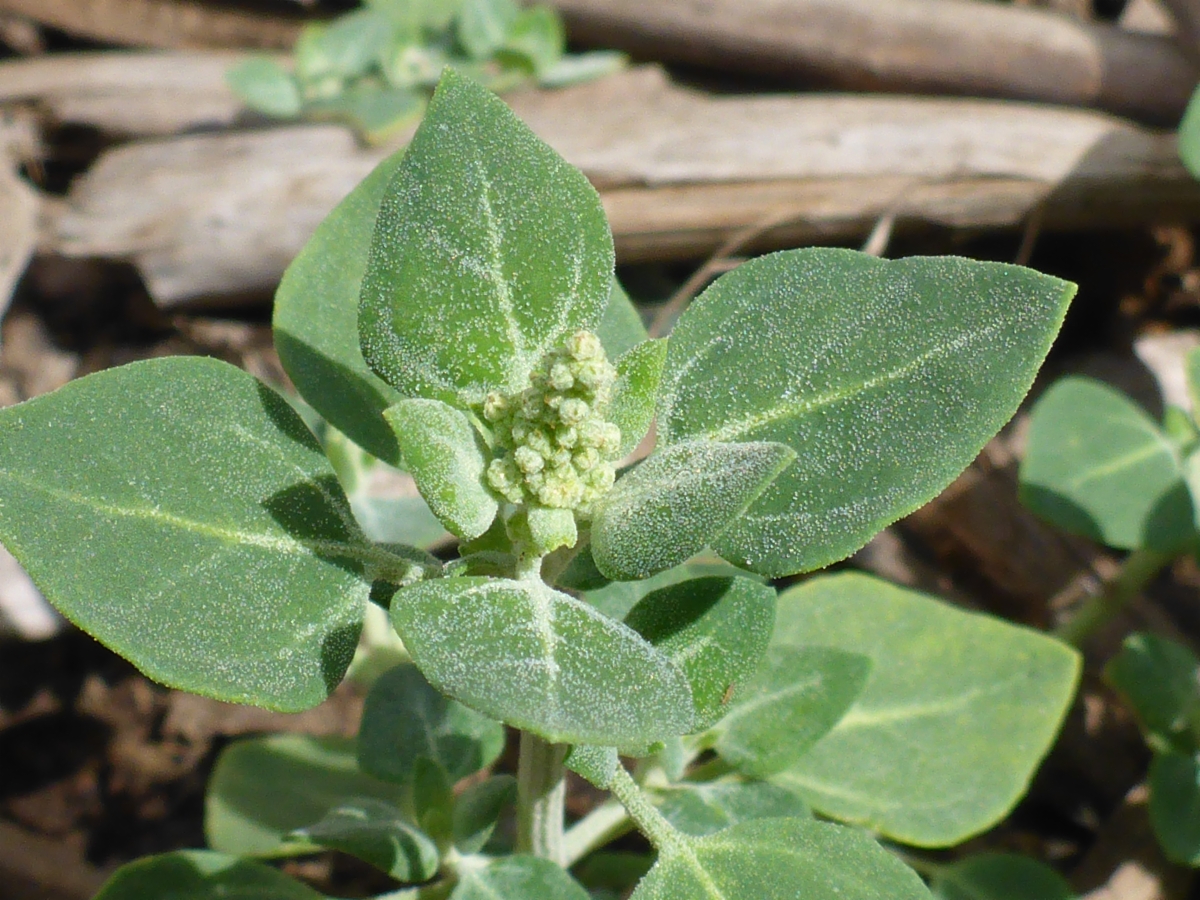The image captures a newborn green plant illuminated by the bright sunlight. Central to the photo is the plant, adorned with medium to large teardrop-shaped leaves that exhibit lighter green veining. The leaves appear to be dusted with a white residue or dew. Toward the upper middle of the plant, the leaves gradually shrink in size, culminating in a cluster of small green buds surrounded by three thin leaves. Just beyond the buds, four slightly larger leaves can be seen, also bearing the same white residue. The scene is set outdoors with fallen logs and other vegetation softly out of focus in the background. The logs have sunshine reflecting off of them, creating a play of light and shadow, and the overall color palette is a natural mix of greens and browns, typical of a sunlit, wooded area.